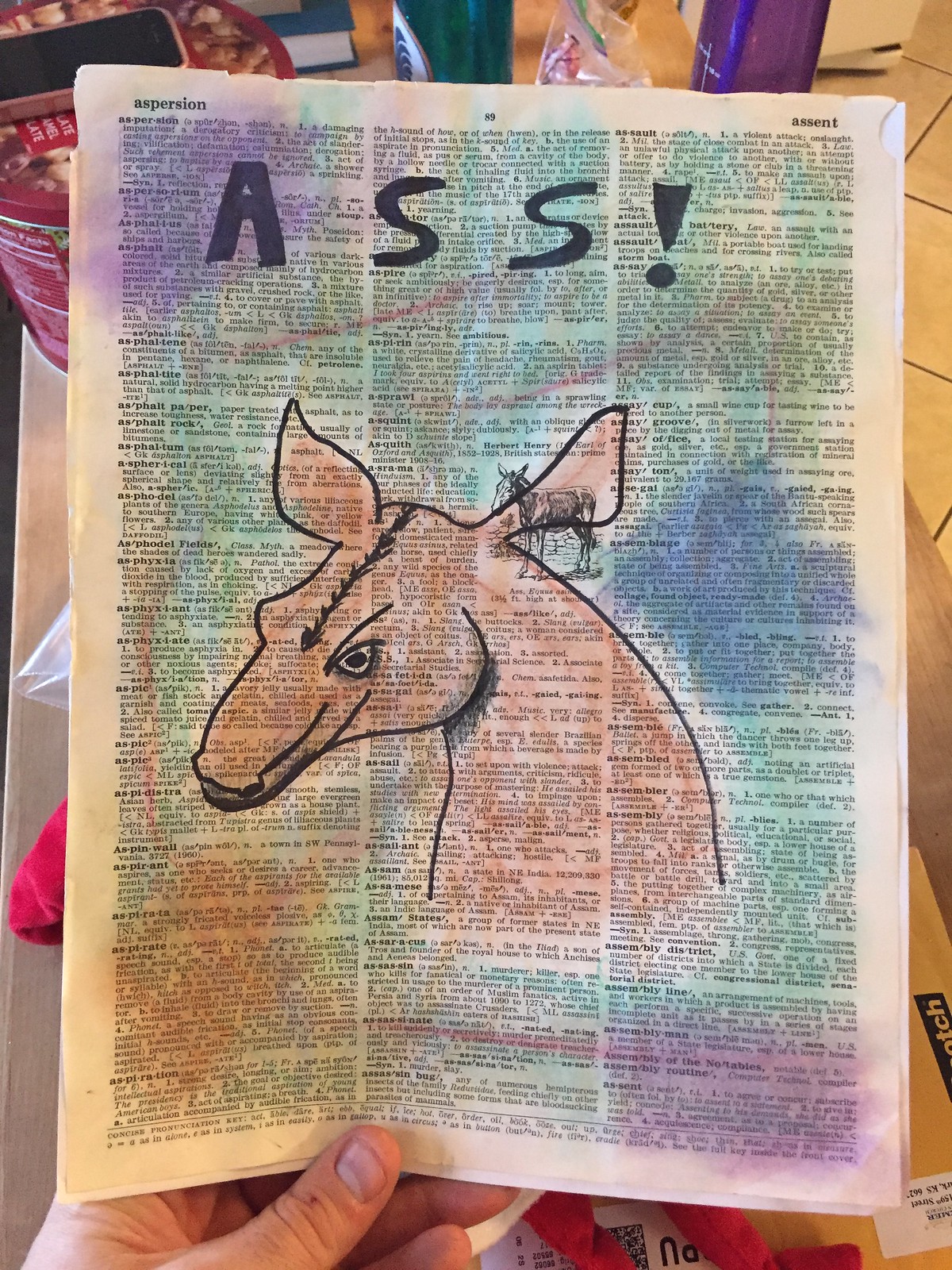This photograph captures a vividly altered page, seemingly torn from a book or magazine. Dominating the bottom of the image is a hand holding the page, its thumb clearly visible. The page itself is a chaotic canvas of vibrant colors, featuring smudges and blobs of purple, green, orangey-tan, and blue. At the center, someone has scribbled the word "ass!" in bold black font. A menacing illustration of a donkey, with an intense expression, dominates the scene. The donkey's distinct features include pointed ears with a strip of black fur running down its head, a sinister single eye, and flared nostrils. Intriguingly, within one of the donkey's ears, there appears to be an inset image of what looks like another donkey or possibly a horse, shaded in brown and black. Every detail on the page suggests a deliberate and imaginative modification of its original content.